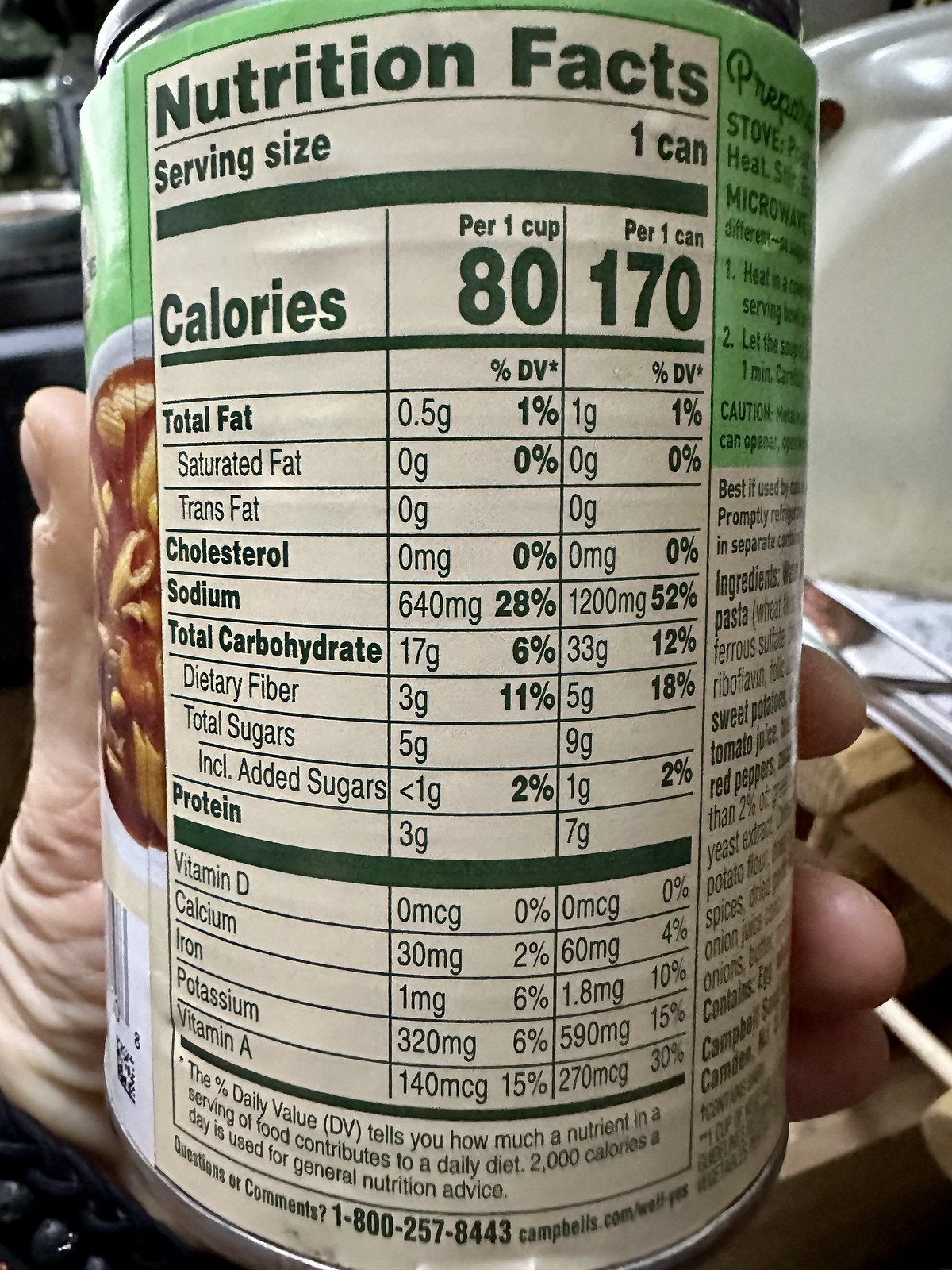In this close-up photograph, an elderly, light-skinned left hand, noticeably wrinkled around the thumb, is holding a tin can with a predominantly green top and a tan nutritional label, bordered by green text. The label includes detailed nutrition facts like serving size (one can), calories (80 per cup, 170 per can), and various nutrient amounts. The can possibly contains soup, depicted by a photo of pasta in a tomato-like red sauce on the left. Curving around the right edge of the can, cooking instructions are visible, mentioning stove and microwave options. A web address appears at the label's bottom. The can is brand identifiable as Campbell’s, and although the surrounding background is blurred, it includes a cream-colored wall and some stacked items.